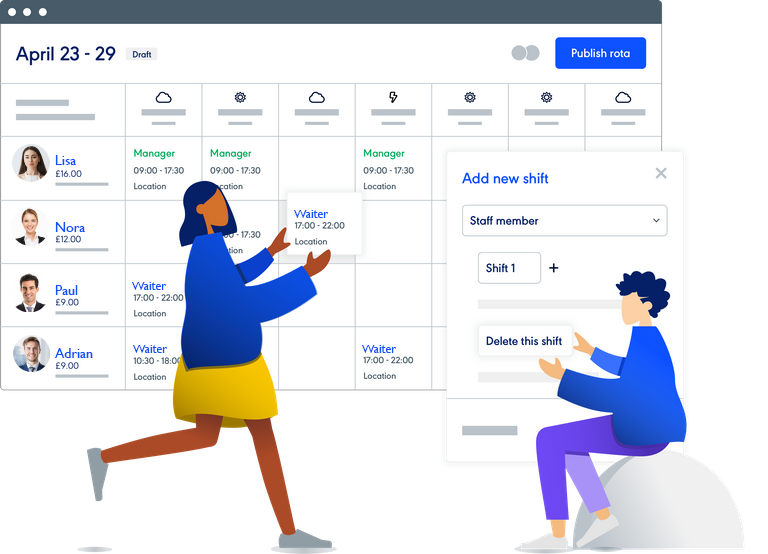"Screenshot of a scheduling calendar interface designed for a server management system. The top portion of the screen features a dark gray stripe typical of a Chrome browser, complete with three dots on the right side. Indicating the time frame of interest, the header displays 'April 23rd to 29th' along with the word 'Draft.' On the far right, a prominent blue button labeled 'Publish Rota' suggests the final step in finalizing the schedule.

The calendar is organized into multiple columns, with the leftmost column showing pictures and names of servers and managers. Seven additional columns are visible, each adorned with icons, though the text beneath them is grayed out and currently illegible. Illustrating user interaction, the screen includes a stylized cartoon of a woman placing a shift card into the calendar. The card she is handling states 'Waiter 1700 to 2200' and includes a section for the location beneath it.

Lower on the screen, another cartoon figure, a man sitting on a rock, appears in front of an overlaid box that reads 'Add New Shift.' This box has a dropdown menu labeled 'Staff Member' and another section marked 'Shift 1' with a plus sign adjacent to it. The cartoon man is also holding a button labeled 'Delete This Shift,' adding to the interface's user-friendly and interactive design."